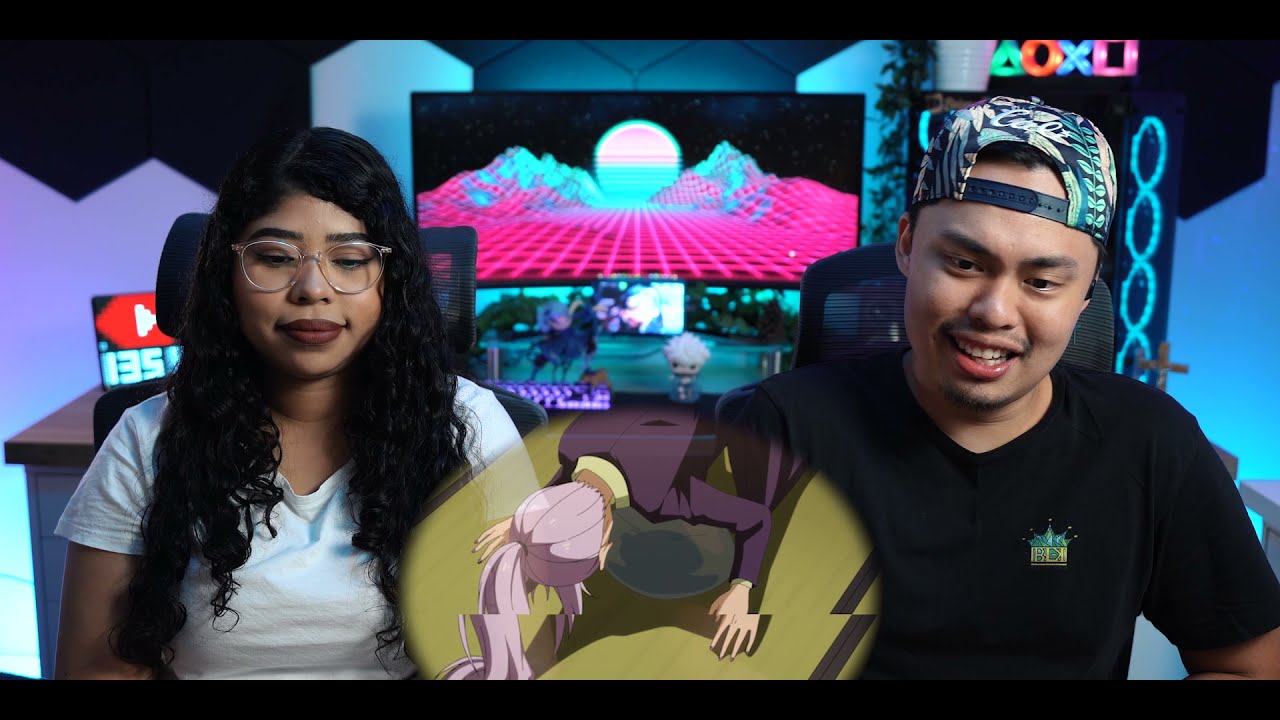The image appears to be a still from a YouTube video or a live stream featuring two individuals reacting to a scene from a cartoon or anime. On the left, a woman with dark skin, possibly Latina or African-American, and long wavy black hair, wearing a light green t-shirt, looks towards the screen. On the right, a man who appears to be Filipino, with dark skin and wearing a black t-shirt and a backwards hat adorned with green leaves, also directs his gaze at the screen. Between them, a superimposed circular image of an anime-style character bowing is visible. The background showcases a computer or TV monitor displaying a futuristic screensaver with a pink grid floor, mountains, and a sun rising in the distance. Additionally, the room features a desk on the left side of the woman with some action figures placed on it, further enhancing the decorative setup. The overall ambience indicates they may be recording a video or live streaming their reactions in a casual, well-decorated environment.